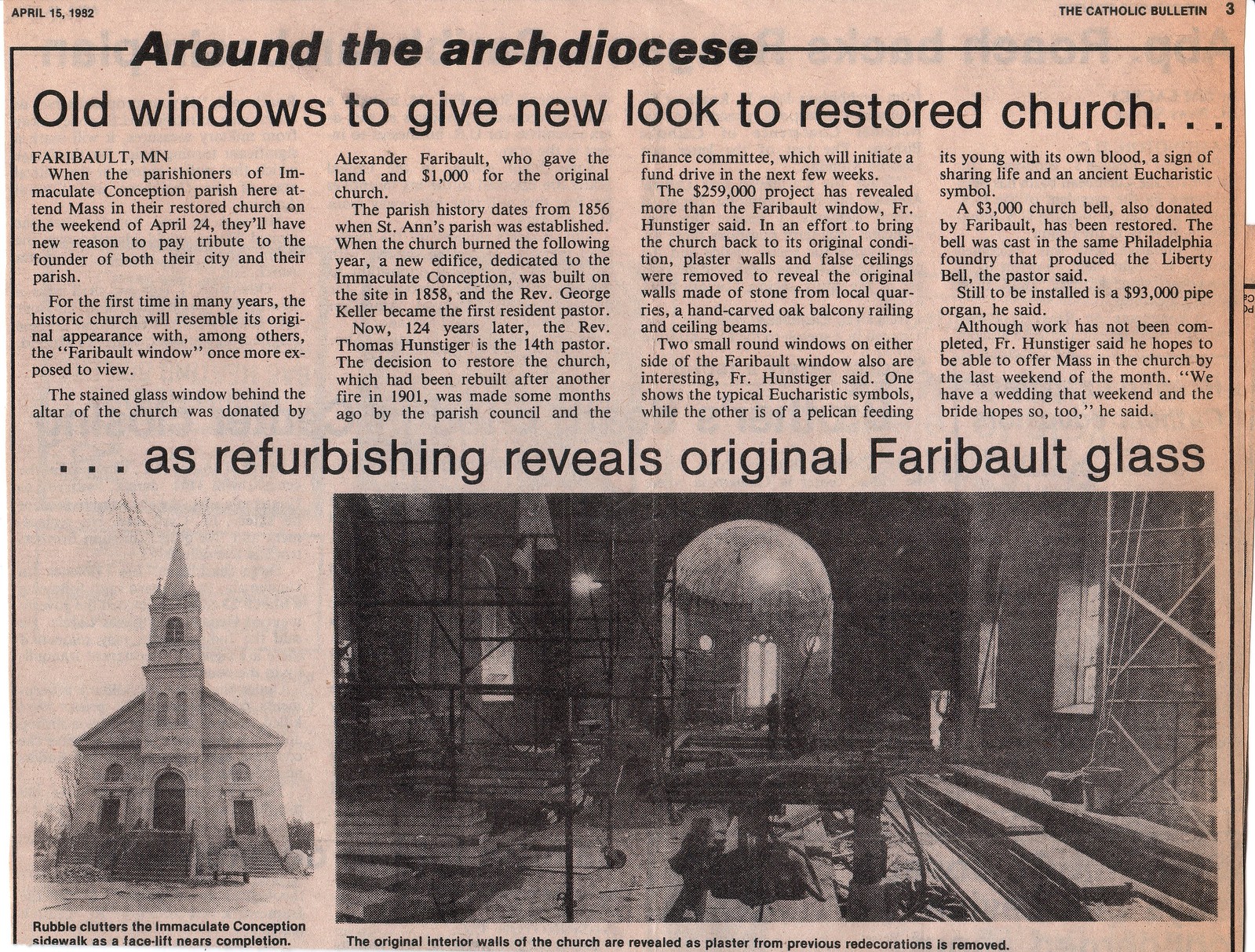This is a newspaper clipping from "The Catholic Bulletin" dated April 15, 1982, focused on the refurbishing of the Immaculate Conception Parish Church in Faribault, Minnesota. The headline reads, "Around the Archdiocese, Old Windows to Give New Look to Restored Church," highlighting the restoration efforts aimed at revealing the church's original stained glass. Beneath this is another headline stating, "As Refurbishing Reveals Original Faribault Glass." The article details that parishioners will attend Mass in the restored church on April 24th, coinciding with an homage to the founder of both the city and the parish. The bottom headline reads, "Rubble Clutters the Immaculate Conception Sidewalk as a Facelift Nears Completion." Accompanying the article are two photos: one shows the church’s interior filled with scaffolding, piles of boards, tools, and workmen, indicating ongoing renovation. The caption under the photo notes, "The Original Interior Walls of the Church are Revealed as Plaster from Previous Redecorations is Removed."